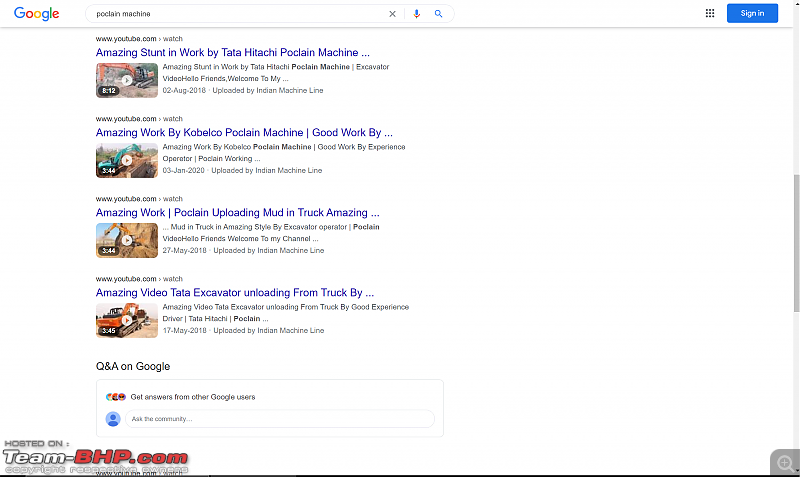A Google search results page is displayed, showcasing the iconic Google logo in its colorful typography. The exact search query typed in the search bar is illegible due to small text size. Prominent results include several intriguing entries such as "Amazing stunt in work by Tata Hiyachi Poclain Machine," "Amazing work by Kabal Co. Poclain Machine," "Poclain uploading mud in truck," "Amazing," and "Amazing video Tata Excavator unloading from truck by something." A watermark on the image reads "hosted on team-bhp.com," indicating that the screen capture was made and possibly found on the automotive forum team-bhp.com.